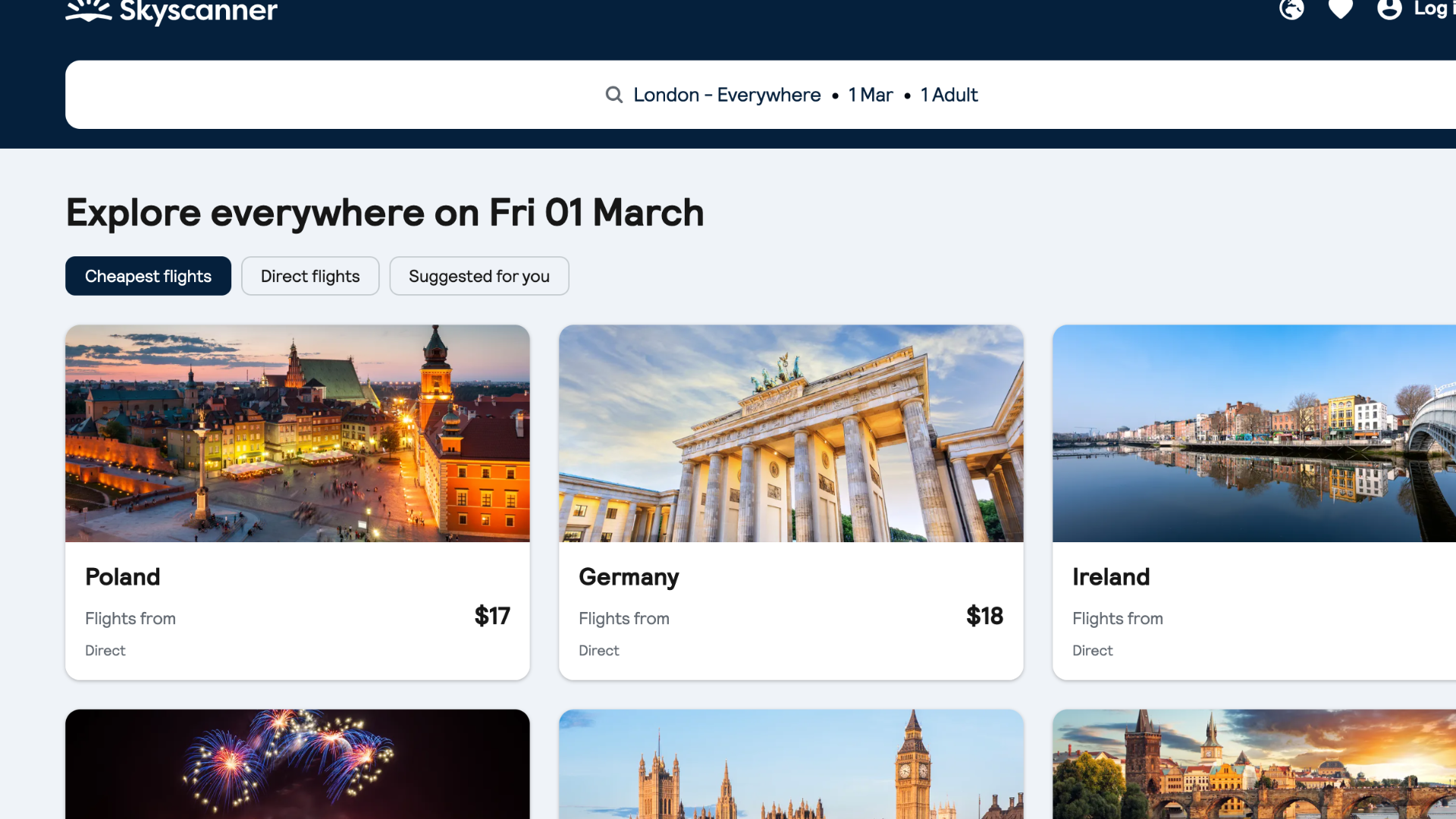The image features a navy blue border at the top with a white, sunrise-style logo on the upper left corner, labelled "Sky Scanner" in white text. In the upper right corner, there are three icons: a globe, a GPS-style dot, and a profile icon, positioned before the partially visible word "log," likely for "login."

Below the border, there is a white search bar area with a magnifying glass icon and the text "London Everywhere, 1 Mar, 1 Adult." Beneath this, a section with a white background and bold black text reads, "Explore Everywhere on Friday, 01 March." Below this, three categories are listed: Cheapest flights, direct flights, and suggested for you, with the "Cheapest flights" option highlighted.

The bottom section of the image displays several thumbnail images of stunning city skylines. The first thumbnail depicts Poland, with the text "Flights from $17, direct." The next thumbnail features Germany, stating "Flights from $18, direct." The third thumbnail is of Ireland, showing "Flights from" and "direct," but the price is cut off.